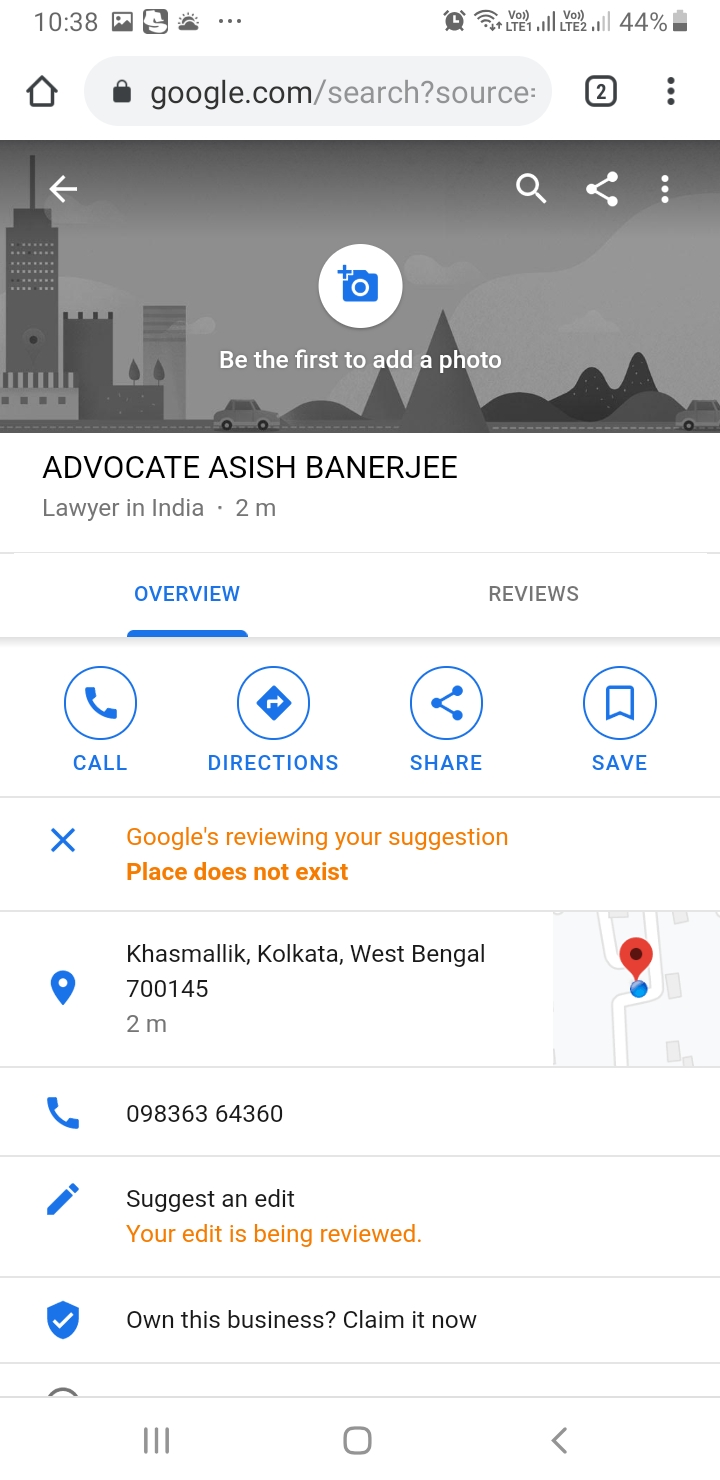The screenshot captures a mobile phone display at 10:38 AM, with various icons visible, including a 44% battery charge indicator. At the top of the screen, the home icon and URL bar are present, showing the user is on a page with the URL "google.com/search?source," indicating a Google search. 

Below the URL bar, there is an option to add a photo, marked by a camera icon and the text "Be the first to add a photo." Beneath this, bold black text reads "Advocate ASISH BANERJEE," followed by the description "Lawyer in India," and indicates the person is two miles away.

The screen displays an 'Overview' section, highlighted in blue to show it is currently selected, with the options 'Overview' and 'Reviews' available. Below this navigation bar, there are icons for 'Call,' 'Directions,' 'Share,' and 'Save.'

Additional information includes a message in orange text stating, "Google is reviewing your suggestion. Place does not exist." The displayed details continue with an address and phone number. At the bottom, options to "Suggest an edit" and "Do you own this business? Claim it now" are available.